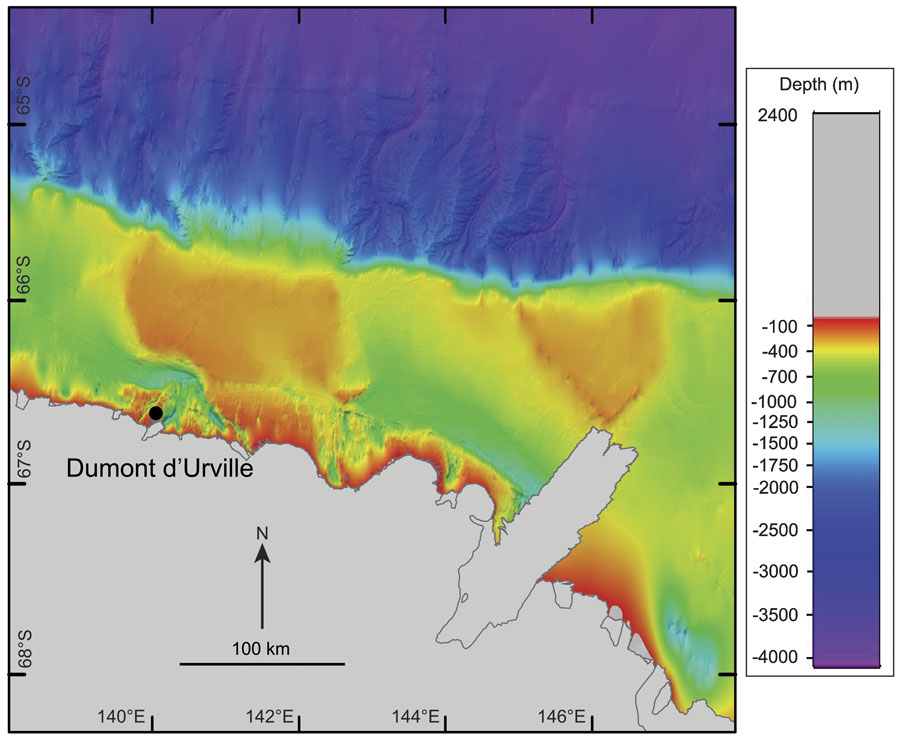This image features a detailed map illustrating water depths off the coastline near Dumont d'Urville. The lower portion of the map depicts the landmass, with a noticeable coastal feature extending outward. The water depths are represented by a spectrum of colors: deep blue indicates depths reaching up to 4000 meters, while green, yellow, red, and lighter blue denote shallower areas as the depths decrease closer to the shore. Coordinates along the bottom of the map range from 140 degrees to 146 degrees east, and from 67 degrees to 68 degrees south on the left. A north-pointing arrow indicates the orientation, and distance is marked by a 100-kilometer scale. A chart on the right-hand side deciphers the color-coded depths, aligning with the various shades seen across the map.